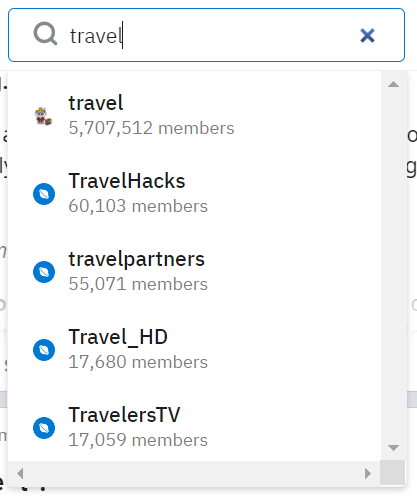The image displays a search interface prominently featuring a large search bar at the top with the word "travel" entered into it. The search bar is white with a blue outline, and an 'X' icon on the right end allows users to clear the search. Below the search bar, a dropdown menu lists various travel-related groups and the number of their members. The list includes:

1. **Travel** - 5,707,512 members
2. **Travel Hack** - 60,103 members
3. **Travel Partners** - 55,071 members
4. **Travel_HD** - 17,680 members
5. **Travelers TV** - 17,059 members

Each group is accompanied by blue icons, mostly depicting a white planet with rings, symbolizing travel or global exploration. The first icon, however, differs and appears as an animal avatar wearing clothes, similar to typical Reddit avatars. The interface overlays a partially visible page in the background, revealing only fragments of letters and some indistinct gray and black areas. The color scheme for the entire image includes shades of brown, yellow, blue, white, gray, and black.